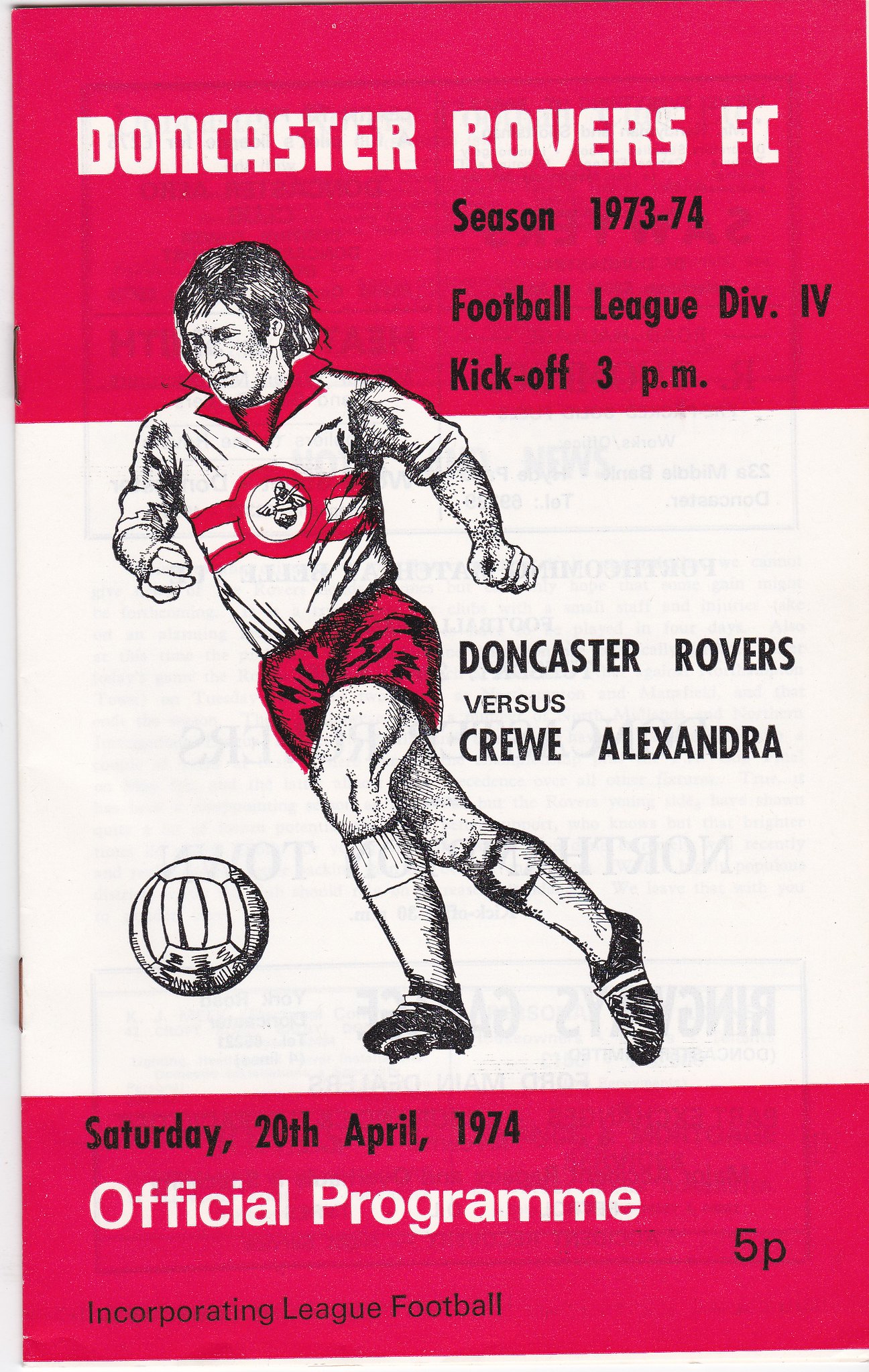This is an image of the front cover of an official program for the Doncaster Rovers Football Club. The booklet, from the 1973-1974 Football League Division 4 season, is structured vertically and bound with two staples on the left-hand side. The top and bottom thirds of the cover are dark red, with the middle section in white. At the top in bold white print, it reads "Doncaster Rovers FC," followed by "Season 1973-1974" in black. Beneath that, also in black, it states "Football League Division 4, kickoff 3 p.m." The center features a black, white, and red drawing of a soccer player in a white shirt with red shorts, poised to kick a ball. Next to this image, the text in black reads "Doncaster Rovers vs. Crewe Alexandra." In the bottom red section, the date "Saturday, 20 April 1974" is printed on the left, with "Official Program" in bold white print in the center, and "Incorporating League Football" in black at the lower left corner. The cost of the program is listed as "5p" for five pence, indicating it is British. The overall color scheme is dull red, black, and white.